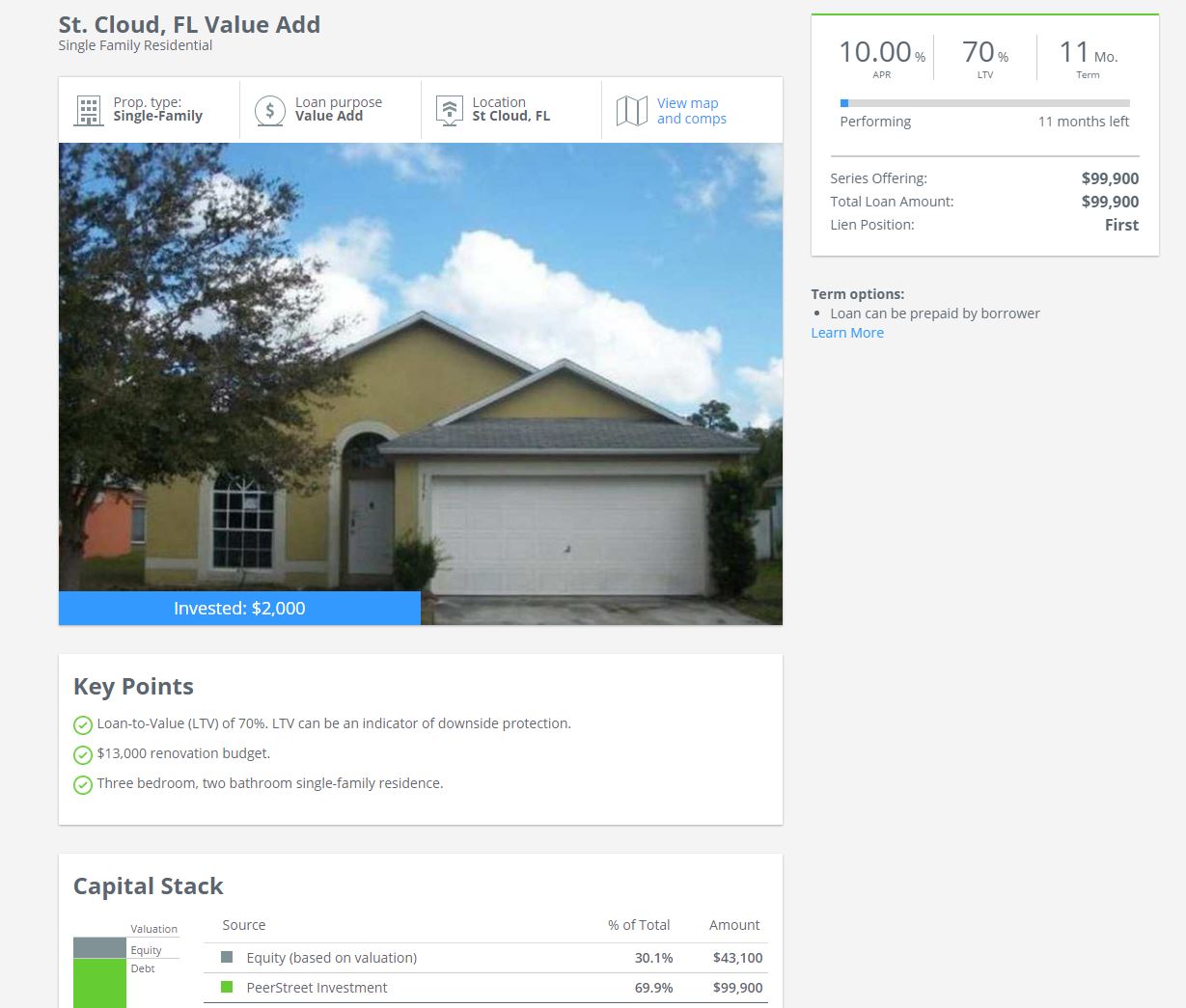**Detailed Home Listing Caption for St. Cloud, Florida Property**

This image is a detailed screenshot from a home listing in St. Cloud, Florida, showcasing a single-family residential property with value-add potential. The background is a muted grayish color. 

At the top left corner, bold text reads "St. Cloud, Florida, Value Add," and beneath it, in smaller text, "Single Family Residential."

The central portion of the screenshot prominently features a home listing. Key details are displayed in four columns:

1. **Property Style**: Single Family
2. **Loan Purpose**: Value Add
3. **Location**: St. Cloud, Florida
4. **Links**: View Map and Comps

Below these columns, there is an image of a daytime exterior view of the house, against a backdrop of clouds. The house is dark yellow, single-story with a two-car garage.

The image contains additional information:
- **Investment**: $2,000
- **Key Points**:
  - Loan-to-Value (LTV) of 70%, indicating a lower risk of loss on the investment
  - $13,000 allocated for renovation 
  - Three bedrooms and two bathrooms

Further details include a visual representation of the "Capital Stack" through a graph. The graph consists of green and gray sections, showcasing equity and debt distribution.

To the right of the graph:
- **Equity-Based Valuation**
- **Pure Street Investment**, indicating the investment type and platform.

This detailed layout offers a comprehensive overview of the property, highlighting key investment and structural details for potential buyers and investors.